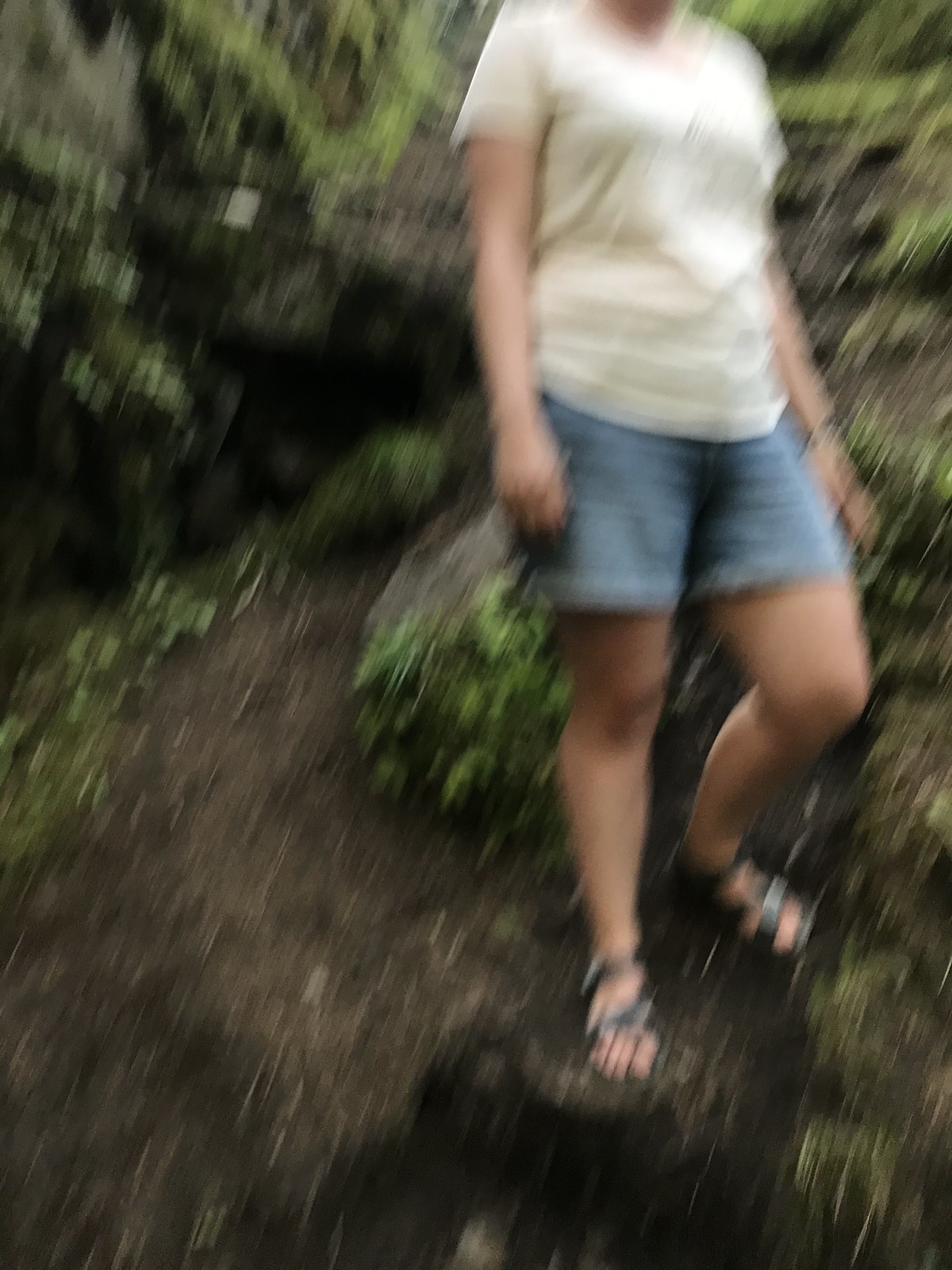The photograph depicts a blurry image of a woman walking through a forest or rocky outdoor area, characterized by abundant green shrubs, foliage, and grasses. The path she walks on appears to be dirt-covered and possibly damp, suggested by the presence of what looks like black rock and an overcast sky. The woman, who is of medium build, is dressed in a short-sleeved white or cream-colored t-shirt, blue denim shorts that come about four inches above her knee, and black sandals resembling Birkenstocks. She has either a bracelet or a watch on her left wrist. The photo seems accidental and taken hastily, perhaps with a phone camera, as her head is not visible, adding to the overall blur and lack of focus in the image.